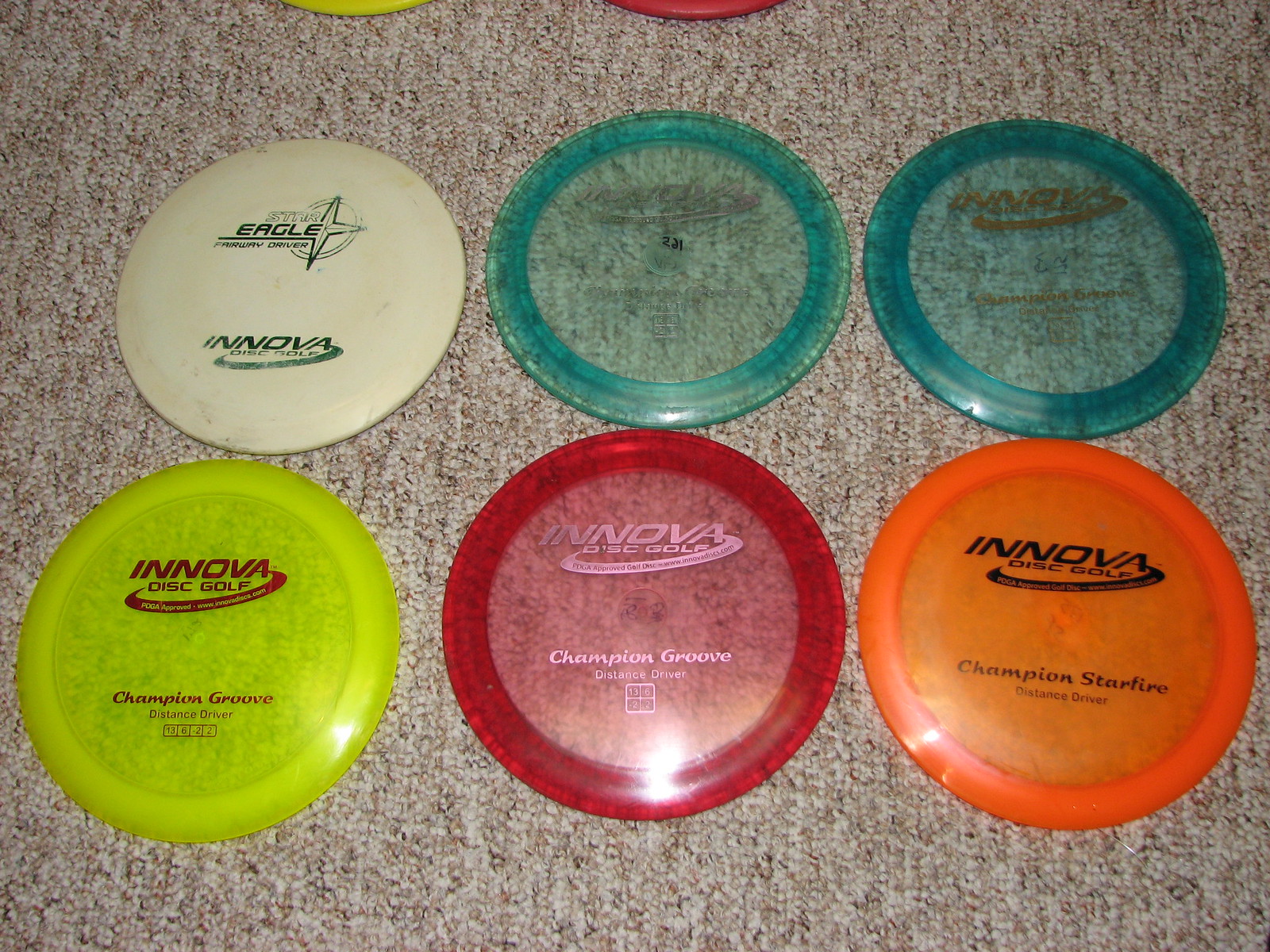The image captures six well-used frisbee golf discs neatly arranged in two rows on a tightly woven, variegated carpet with a color palette of whitish gray interspersed with tan and dark brown speckles. The bottom row features a bright yellow disc with "Innova Disc Golf" inscribed in red lettering, followed by a translucent red disc of the same brand, and a bright orange disc labeled "Innova Disc Golf Champion Starfire Distance Driver." In the top row, from left to right, there's a heavily worn white disc marked as an "Eagle Fairway Driver" with a star next to the word "Eagle" and the "Innova" branding, a clearish turquoise-blue disc with indistinguishable writing due to wear, and a slightly darker blue disc also branded by "Innova." Additionally, the top edge of the photo reveals just a glimpse of two more discs—one yellow and one red—peeking into the frame. The consistency in branding suggests a collection predominantly from Innova, featuring models like the Champion Groove Distance Driver and Champion Starfire Distance Driver.